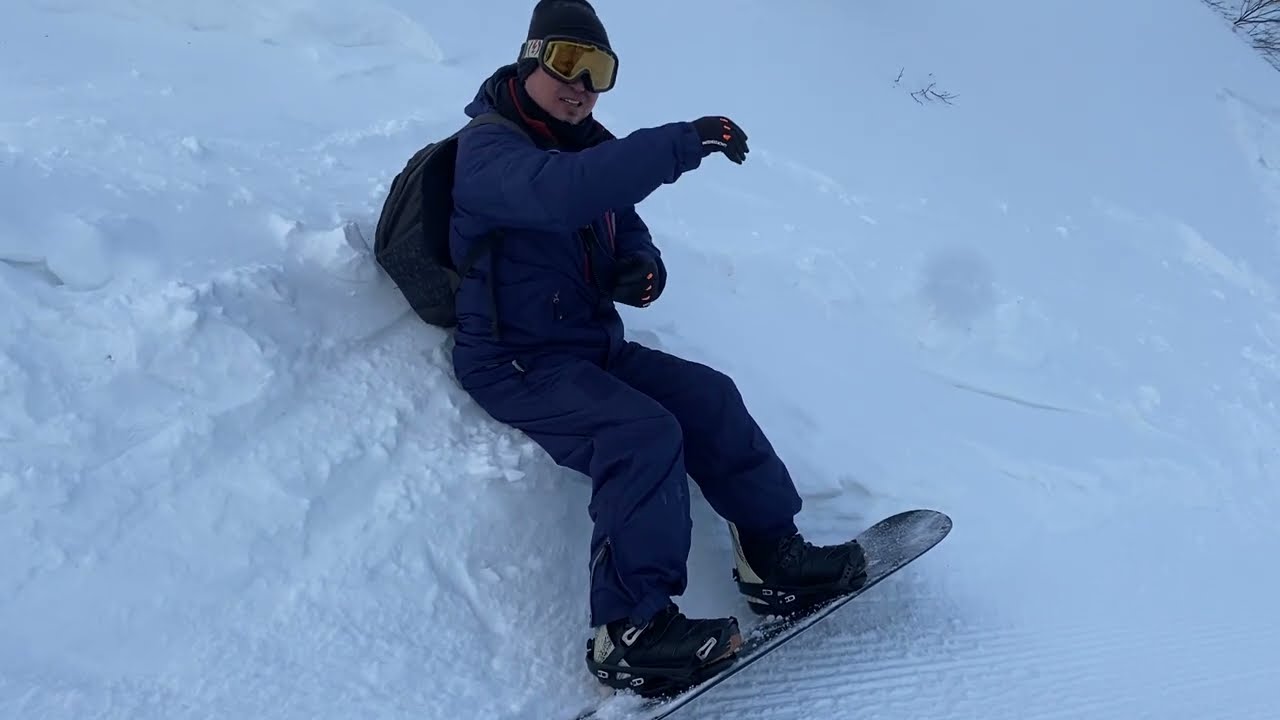The image captures a snowboarder who has fallen or is seated on an incline in the snow. He is wearing a blue snowsuit that covers his entire body, along with black snowboarding boots and black gloves that have white and orange detailing. A black backpack is situated against the snow, and he sports a black beanie along with goggles featuring a yellow tint. His knees are slightly bent, and his snowboard remains fastened to his feet. He has his right arm raised in front of him, possibly stretching or checking for injury, and his expression suggests either a smile or a grimace of pain or annoyance. Snowboard marks form a horizontal line pattern on the snowy slope beside him. The background is predominantly snow-covered with a hint of trees or brush visible in the top corner.